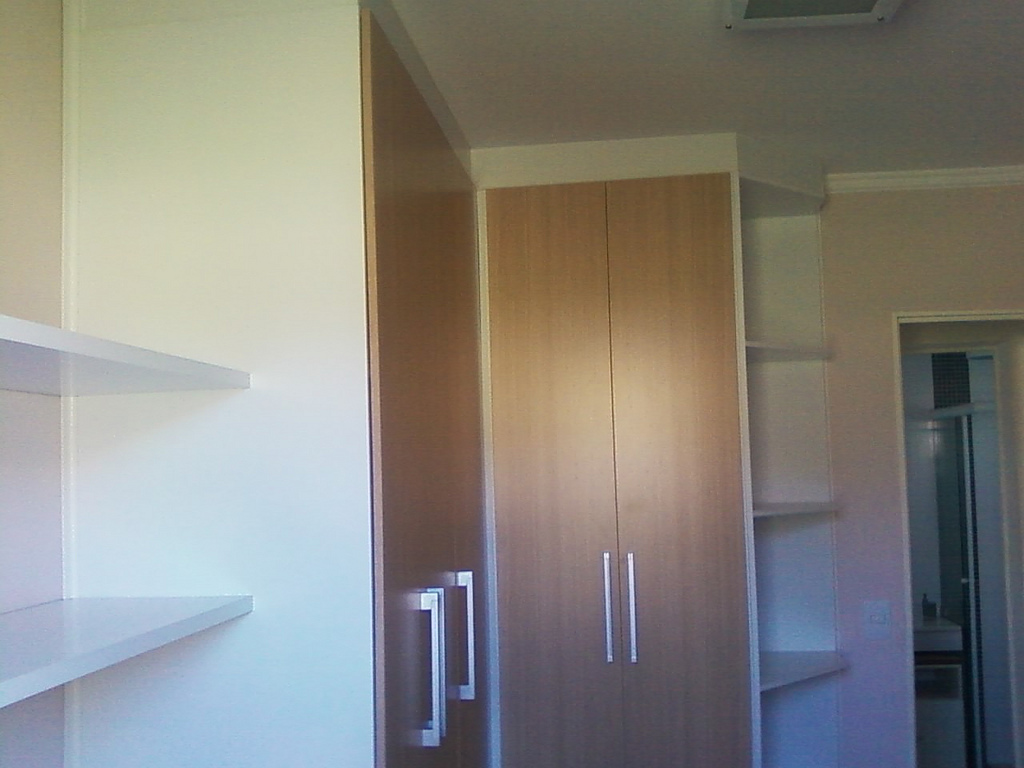This photo shows the interior of a compact room that could be a hotel, apartment, or dorm room. The image quality is somewhat grainy, rendering distant objects slightly blurry, likely due to lower resolution. The left side of the room features a white wall with empty white shelves. Directly ahead are two sets of brown wooden double doors with silver metallic handles, likely closet doors. These doors exhibit visible grain patterns, adding a touch of texture to the scene. To the right of these closets is a corner section with three additional white shelves. Adjacent to this is a pink-painted wall with a white doorframe leading to what appears to be a bathroom. The ceiling is painted white and includes a visible vent. The room is otherwise empty, accentuating its compactness and the light pink hue of the walls, which might suggest it is awaiting new occupants or further furnishing. A light switch is also noticeable on the wall near the doorway.